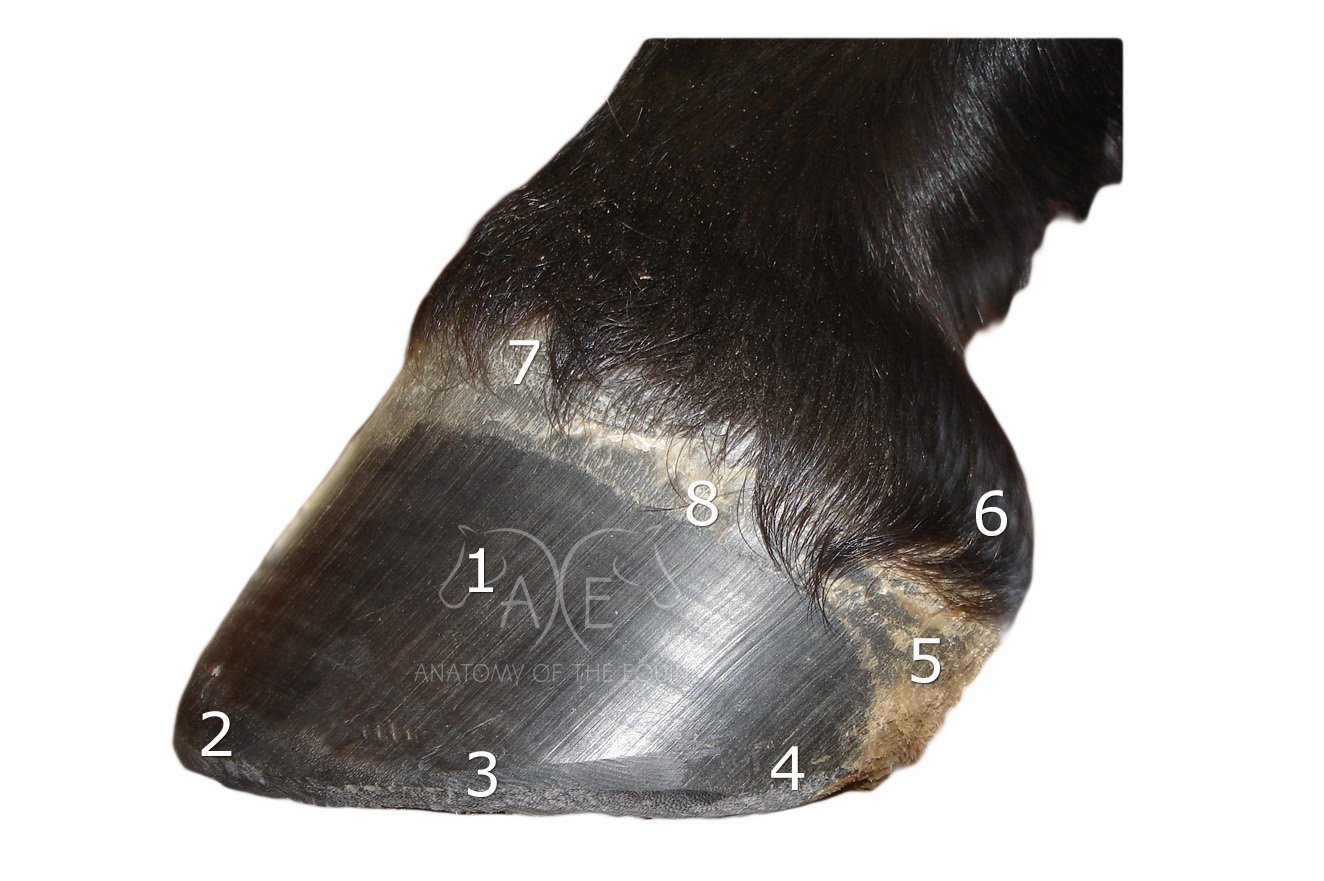The image depicts a zoomed-in view of an animal's hoof, most likely a horse, positioned at a 45-degree angle on a white background. The hoof is partially encased in black, shiny fur that extends slightly up the leg, with the visible section of the leg being lean and not extending far beyond the hoof itself. The hoof material appears gray and has a detailed texture.

Various points on the hoof are labeled with numbers etched or printed on its surface. Number 1 is centrally located on the hoof, while numbers 2, 3, and 4 are aligned along the bottom edge. Numbers 5 and 6 ascend up the side, with numbers 7 and 8 positioned over the top. Additionally, there's a stylish watermark featuring two back-to-back horse heads; one head is labeled with an "A," and the other with an "E," forming a visual emblem between them. Below this emblem, partially obscured text reads "Anatomy of the..." which remains unclear due to a glare.